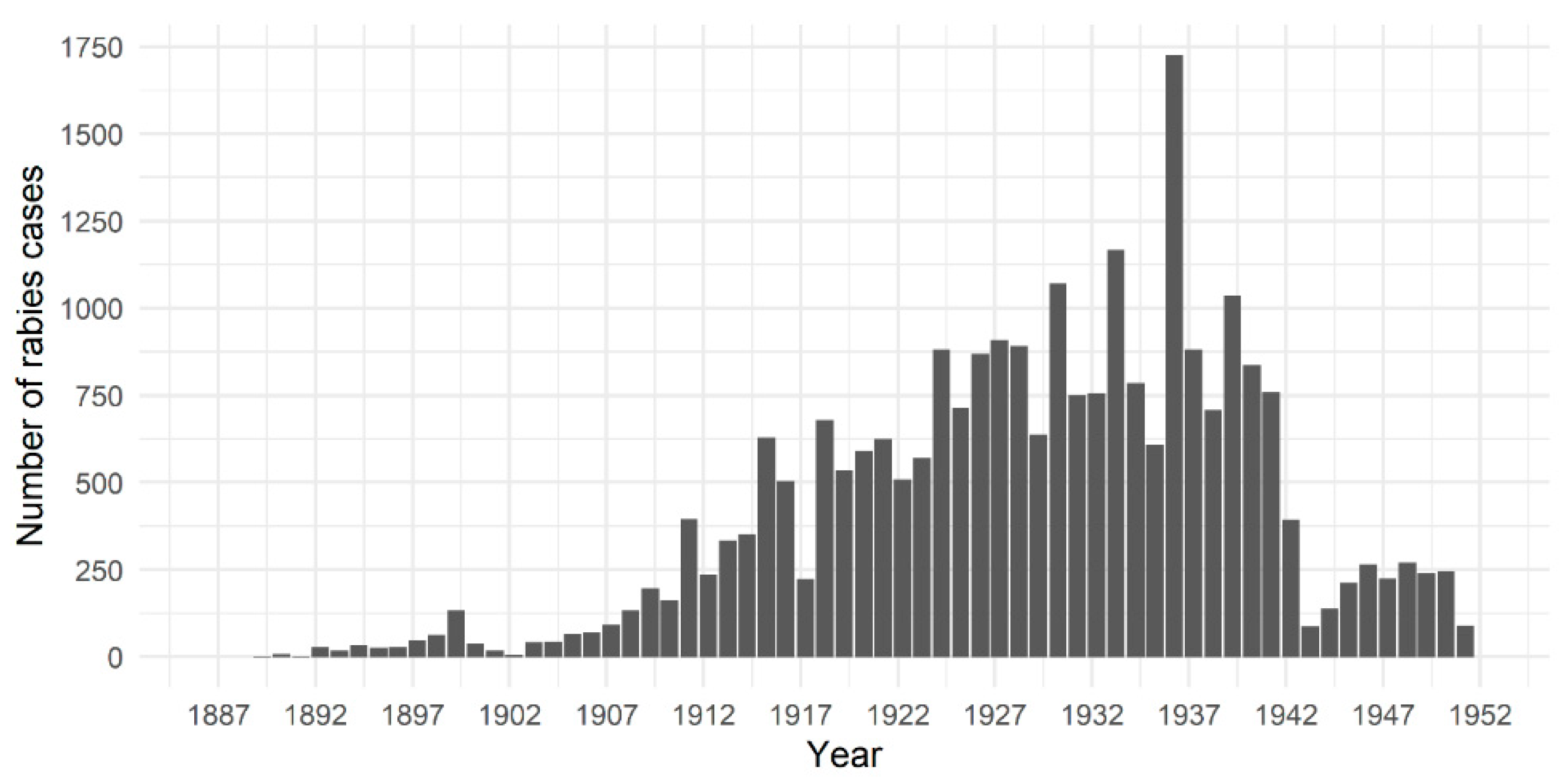This black and white bar chart illustrates the number of rabies cases from 1887 to 1952. The y-axis, labeled "Number of Rabies Cases," ranges from 0 to 1750, with increments of 250. The x-axis, titled "Years," marks years in 5-year increments, beginning at 1887 and ending at 1952. Initially, the chart shows very few cases, but there is a noticeable increase around 1900 with approximately 125 cases. The number of cases continues to rise, peaking around 1936 with almost 1750 cases. After a significant decline in 1943, the chart exhibits a slight increase, then stabilizes to less than 125 cases by 1952.